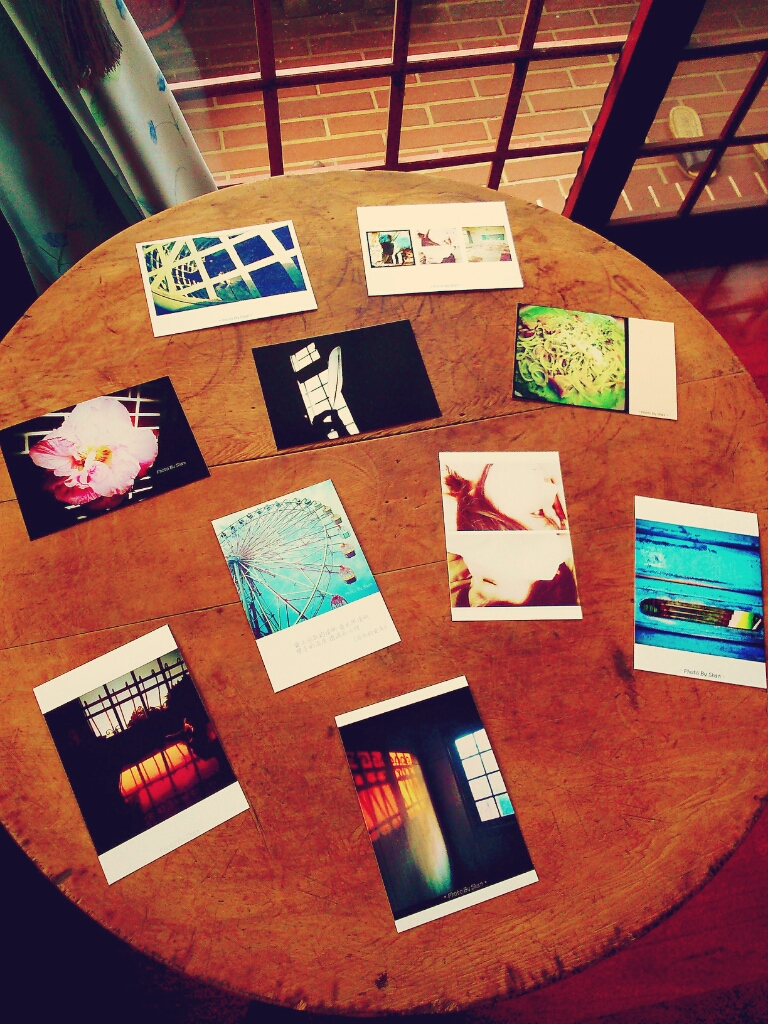In this image, an old, circular wooden table takes center stage, its surface marked by the passage of time with numerous carvings and markings that tell stories of its long history. The focus of the image, however, lies squarely on an eclectic array of photographs scattered across the table. 

At the bottom of the display, a photograph captures a room awash with light, reflected from a window onto the wall. Beside it, a darker image showcases a mysterious-looking gate under dim lighting. To the right, a picture of a swimming pool emerges, though partially obscured and faint, making details hard to discern. Adjacent to this is a very bright image, possibly depicting flames, its clarity overwhelmed by its brightness. 

Continuing around the table, a vivid close-up of a Ferris wheel stands out, easily recognizable among the collection. An image of a delicate pink flower occupies the upper section, exuding a serene contrast to the surrounding photos. Nearby, a photograph captures a hand gently holding a feather, adding a touch of softness to the otherwise varied assortment. Further along, another depiction of a gate appears, contributing to a subtle theme of entranceways.

Completing the array, an image of a peculiar greenish food, which looks like noodles, brings a quirky and whimsical element to the curated ensemble. The seemingly random yet fascinating collection of images invites viewers into a contemplative and visually stimulating experience.